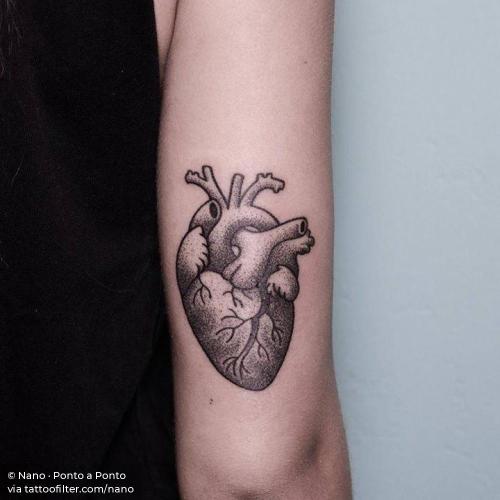This photograph showcases a realistic anatomical heart tattoo situated on the back of a young male's upper right arm, specifically near the tricep area. The black and white tattoo intricately depicts the basic structure of the heart with visible chambers, ventricles, veins, and vessels. The subject is wearing a black tank top, and the image captures the back of his right arm from just below the shoulder to just above the elbow. The tattoo is centered and stands out against the bare skin, approximately an inch above the elbow. The background includes a white wall occupying the right third of the image. Additional text at the bottom left corner reads "via tattoofilter.com/nano."